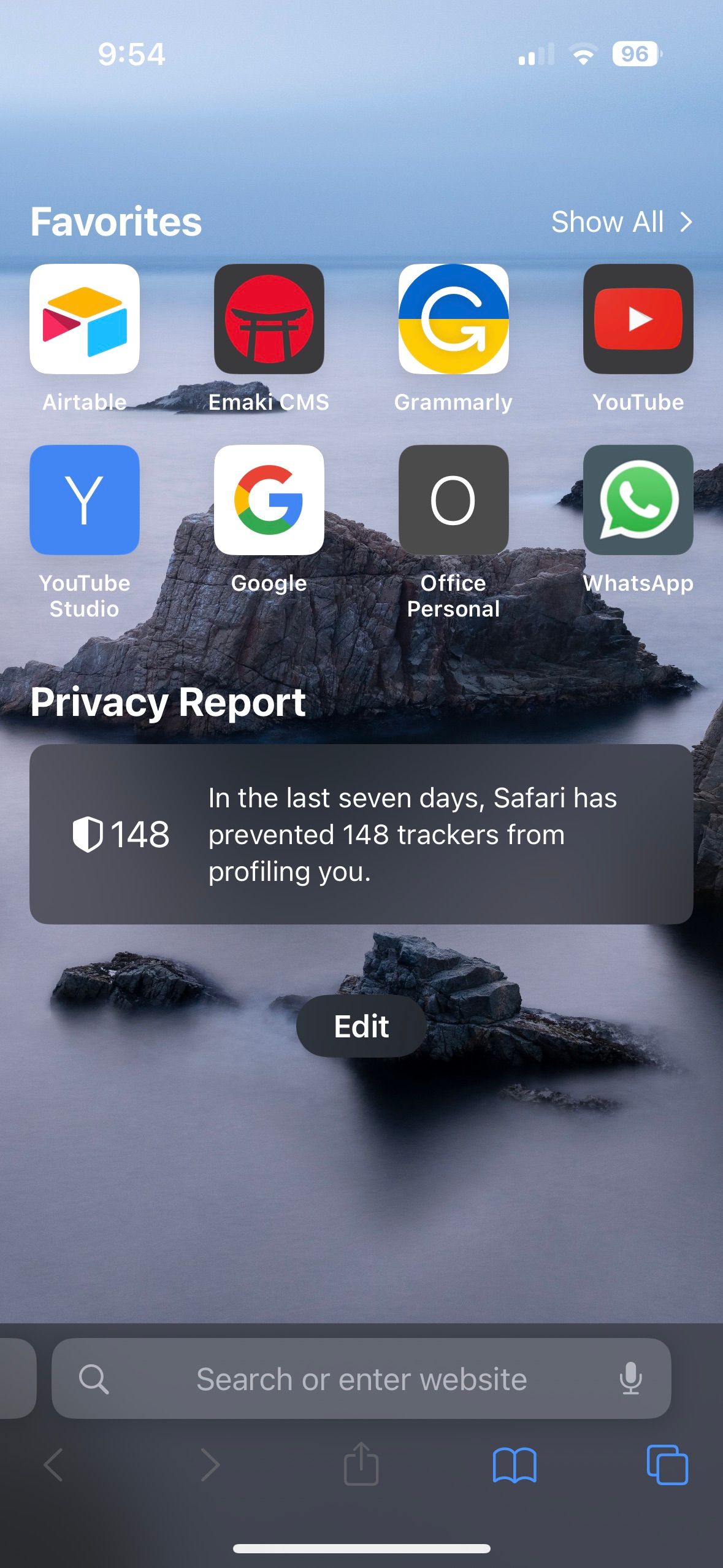The image is a screenshot from a mobile device, showcasing a customized home screen with various UI elements and apps. 

**User Interface and Status Bar:**
- At the top of the screen, the status bar displays crucial information:
  - **Time**: 9:54 AM, shown in white text on the left side.
  - **Signal Strength**: Two out of four bars, indicating moderate signal strength, on the right side.
  - **Wi-Fi Connection**: Two out of three bars, suggesting a decent connection, next to the signal indicator.
  - **Battery Status**: A horizontally positioned icon displaying "96%", indicating a nearly full battery.

**Favorites Section:**
- Under the status bar is a special screen section titled "Favorites" in white text, followed by a "Show All" button with a right-pointing arrow (greater than symbol).
- This section contains two rows of favorite app icons:
  - **First Row**: Airtable, Emac ECMS, Grammarly, YouTube
  - **Second Row**: YouTube Studio, Google, Office Personal, WhatsApp
- All icons are square-shaped and presented in a neatly organized grid.

**Privacy Report Section:**
- Below the favorites, a heading labeled "Privacy Report" is displayed.
- Beneath it, a dark gray rectangle provides privacy information with a shield icon and the number 148 on the left.
- Accompanying text on the right states: "In the last seven days, Safari has prevented 148 trackers from profiling you."
- An oval-shaped dark gray button labeled "Edit" in white text is beneath this information.

**Navigation Bar:**
- At the bottom of the screen is the phone’s navigation bar featuring:
  - **Search Bar**: "Search or enter website," with a magnifying glass icon on the left and a microphone icon on the right.
  - **Navigation Icons**: Includes buttons for previous, next, exit, an open book (likely for bookmarks), and possibly a copy function.

**Background Image:**
- The entire setup is overlaid on a serene background image of dark rocks in a body of water. The scene appears overcast and moody, with gray and bluish tones that convey calmness and tranquility. Most icons obscure the background but the peaceful essence of the image is still perceptible.